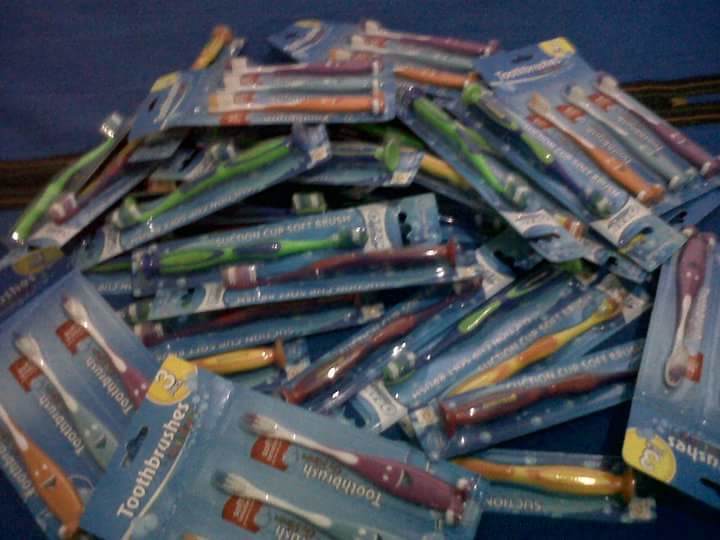This blurry, grainy photo displays a large, chaotic pile of toothbrushes still in their clear plastic packaging, which is strewn haphazardly across a tabletop. Most of the toothbrushes are in packs of three, showcasing uniform colors within each pack, such as maroon, light blue, and orange. Some packs contain individual toothbrushes, particularly in lime green, yellow, or blue, and a few packs contain sets of two. Notably, several packs of three include orange, blue, and purple toothbrushes that feature smiley faces. The text on the packaging indicates "toothbrushes" at the top, along with a number, mostly "three," indicating the quantity within each pack.